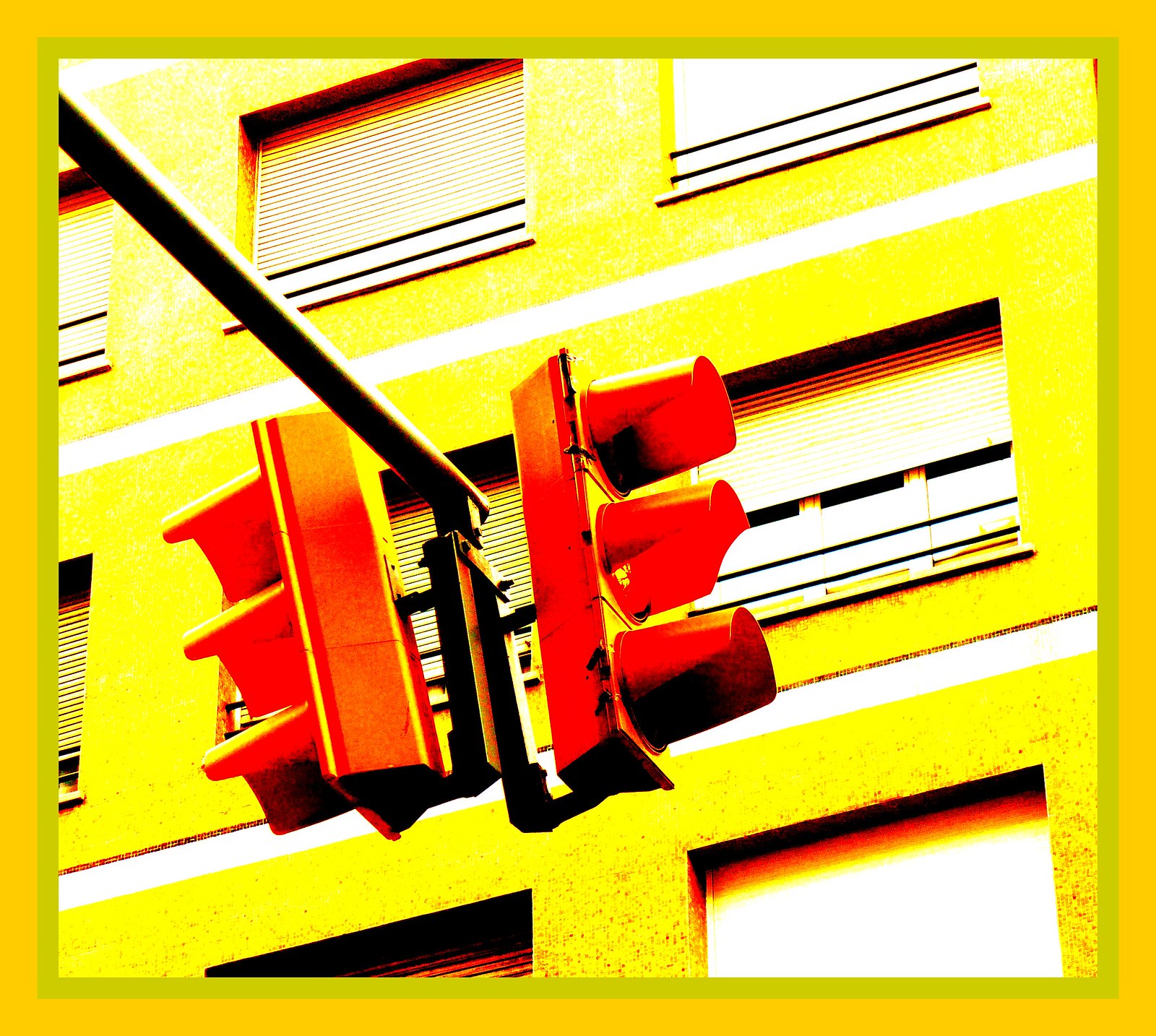In this highly saturated image, we observe two metallic yellow traffic lights mounted on a dark pole. Each traffic light faces an opposite direction, positioned back-to-back with a small black brace connecting them. The traffic lights are vertically aligned with three individual lights in each set. Behind the traffic lights stands a yellow multi-leveled building, resembling a skyscraper. This building features at least three stories and multiple windows, with four windows visible outright—two stacked pairs—and two more partially seen on the left side of the image. The photo itself is square-shaped, framed by an olive green border surrounded by a yellow frame. The overall view appears to be from a low angle, looking upward at the traffic lights and the towering structure in the background.